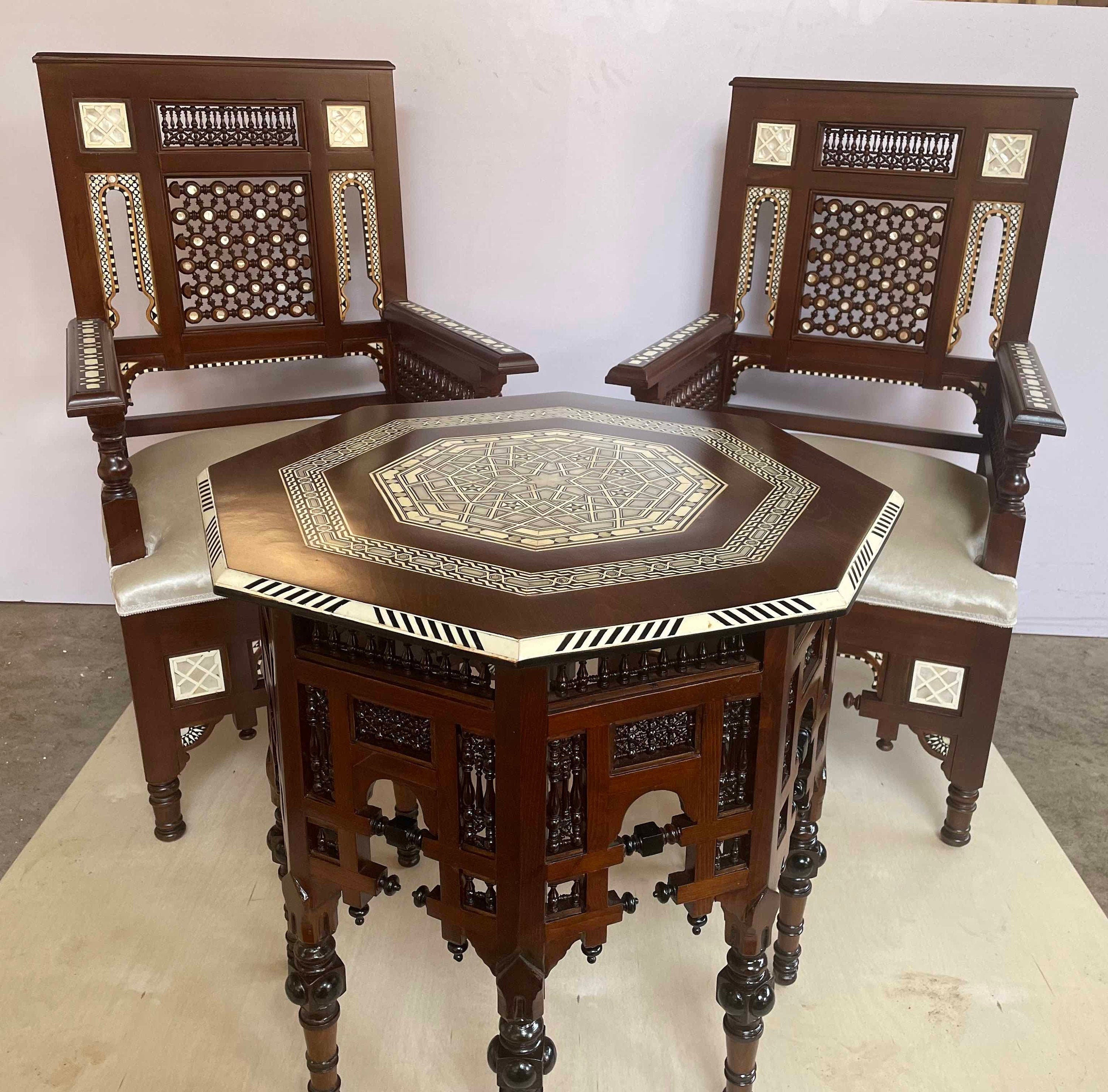In this indoor photograph, which is approximately six inches high and six inches wide, we see a carefully arranged setting featuring a central octagonal table paired with two matching antique wooden chairs. Both the table and chairs sit atop a light brown plywood panel, distinctly placed on a gray concrete floor. The background features a light-colored wall, possibly pink or white, adding a subtle contrast to the setting.

The octagonal table, intricately designed with geometric and perhaps bone inlay patterns, has eight legs and features a criss-cross Celtic-like motif in the center, encircled by beveled edges with horizontal black lines. The wood is a rich dark brown, complementing the elegant latticework along the sides.

The two chairs behind the table are identical, made of the same dark wood and sharing the table's intricate craftsmanship. The chairs boast cream-colored or white satin cushions, with ornate latticework and round elements on the backs and arms, possibly incorporating similar bone designs as the table. The overall antique theme ties all pieces together, creating a harmonious and detailed aesthetic against the contrasting background and floor setting.